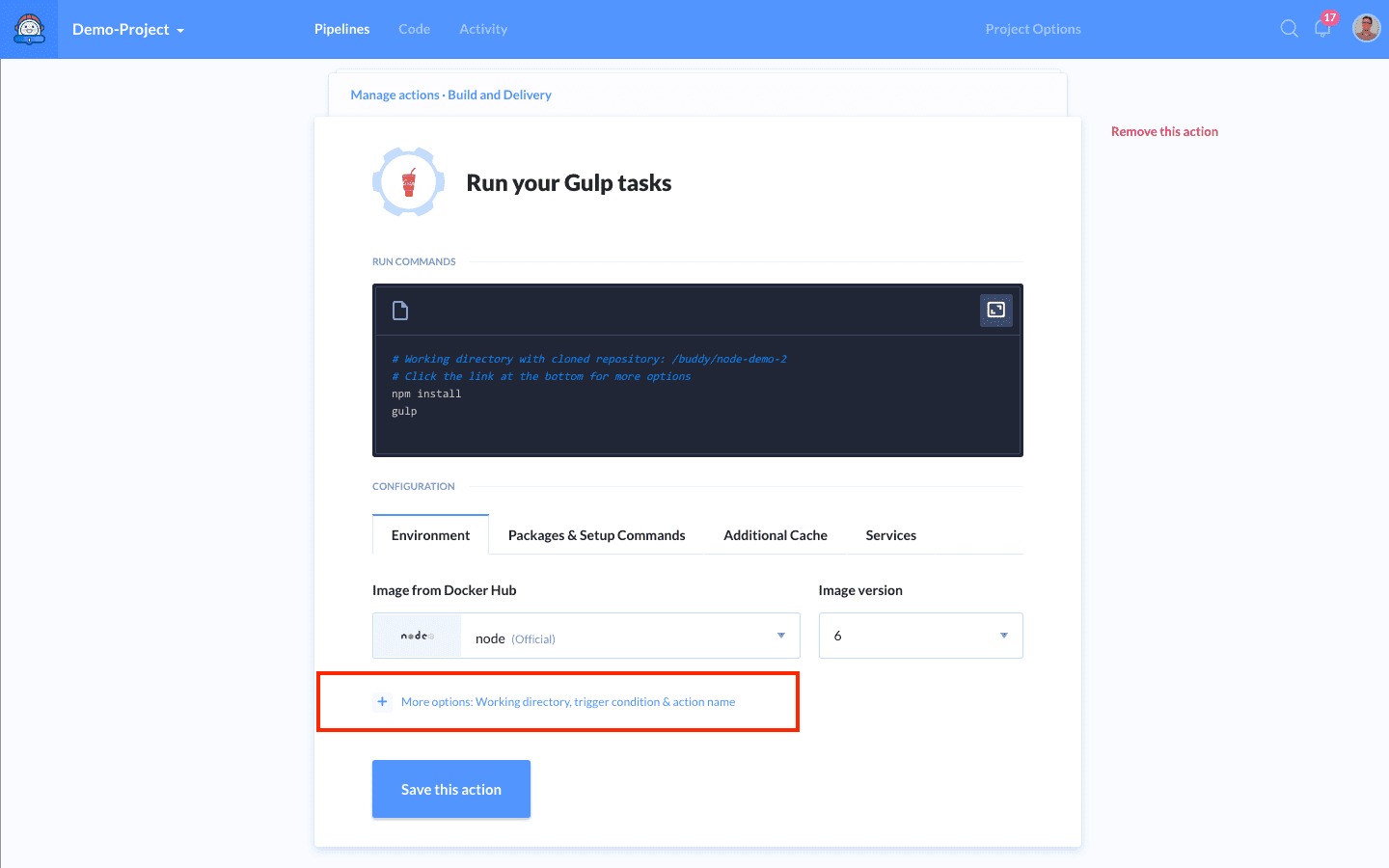This is a detailed screenshot of a web-based platform for software development, titled "Demo Project" a the top left corner. The interface appears to be part of a live demonstration for a project currently in progress. The top navigation bar features several tabs, including "Portfolios," "Pipelines," "Code," and "Activity," with "Portfolios" being the active tab while the others are grayed out. 

Immediately below the navigation tabs, there are sections labeled "Manage Actions," "Build and Delivery," with a prominent "Run Your Gulp Tasks" title highlighted in black text. Adjacent to this title, on the left, is an icon resembling a hexagon enclosing an illustration of a beverage with a straw, possibly representing a tool or feature related to task automation or workflow management. 

The lower portion of the screenshot shows an area displaying code in a structured format, featuring syntax highlighting in blue and white text, indicative of a coding environment. The exact text is indistinct, but the layout and design suggest this platform is tailored for code sharing and collaboration among developers.